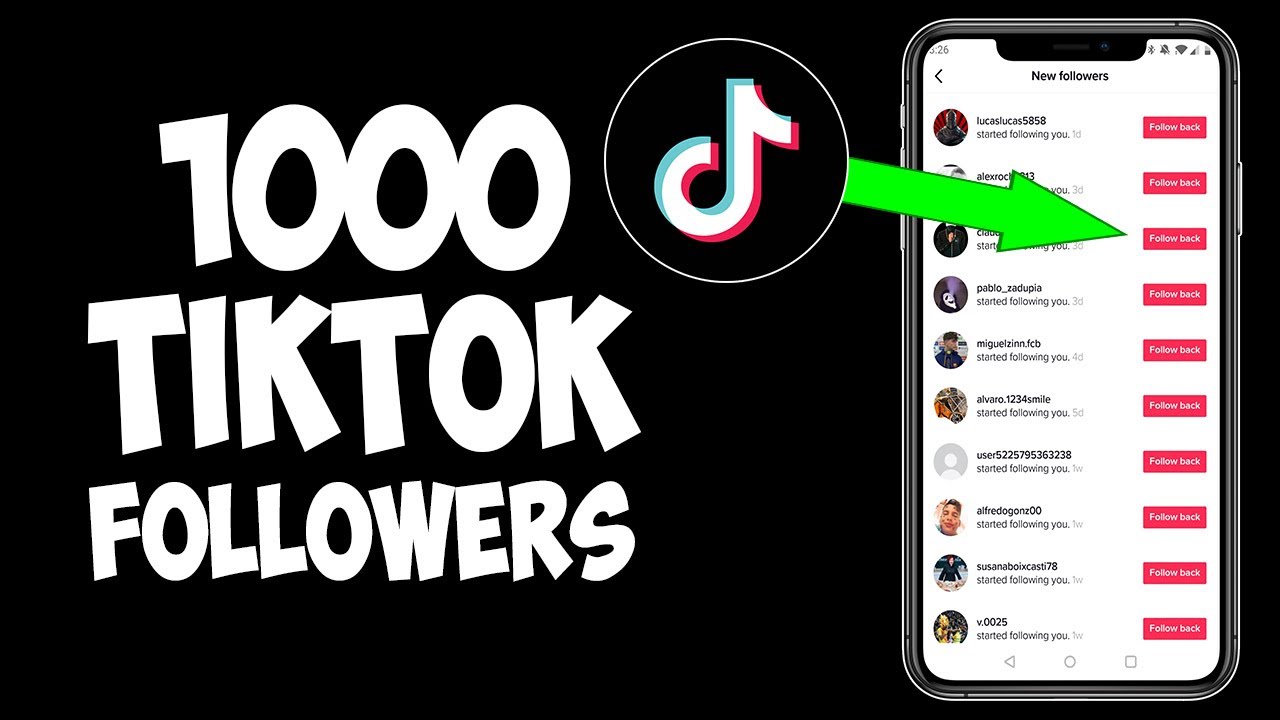This image is a promotional TikTok advertisement. The background is predominantly black, with an eye-catching, large white text occupying about two-thirds to three-quarters of the left-hand side. The text is in a playful, cartoonish font and reads "1,000 TikTok followers." Below this text is a small circle featuring the TikTok logo, accompanied by a bold, green arrow pointing to the right.

On the right-hand side of the image, a simulated iPhone display takes up the remaining one-quarter of the space. The iPhone screen showcases a list of new followers, each entry formatted with the follower's username, followed by the text "started following you." The top username displayed is "Lucas5858," and there are a total of ten new followers listed. Next to each username, a "follow back" button is visible. Most of the follower entries have individual profile icons, with only one showing the default grayed-out avatar. The followers appear to have started following the user within a timeframe of one to seven days.